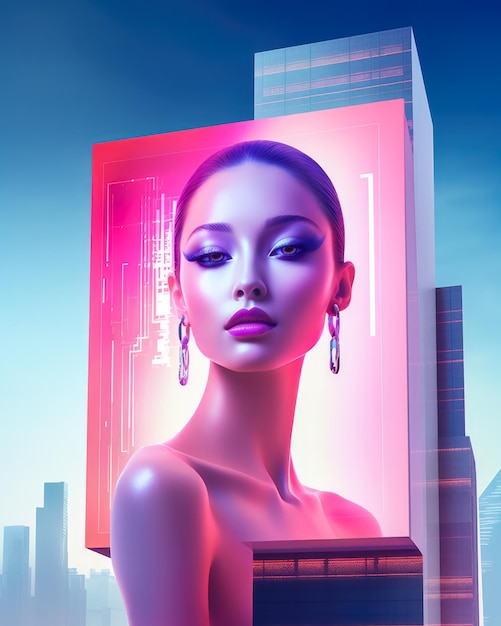An ultra-modern, computer-generated cityscape, bathed in vibrant neon pinks and blues, showcases towering skyscrapers against a futuristic skyline. Dominating the foreground is an enormous digital billboard, resembling a computer screen. The billboard features a striking advertisement with the image of a woman, visible only from the shoulders up. She exudes an enigmatic, artificial allure, characterized by her tight, dark ponytail, and large hoop earrings. Her heavily made-up eyes, adorned in shimmering blue and silver, contrast sharply with her clear skin and glossy pink lips. The woman's appearance suggests she is an AI model, seamlessly blending into the high-tech ambiance of this visionary metropolis.